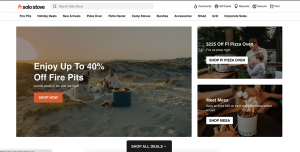A small webpage showcasing various fire pits. The homepage, primarily white with black text and accented with orange elements, displays three small images. The first image features a couple gathered around a cylindrical fire pit on a beach. The second image highlights a promotional banner offering up to 40% off on selected fire pits. The third image includes a child, suggesting family-friendly fire pit designs, though the specifics are unclear due to the image size. Each fire pit appears designed for containing and sustaining fire, showcased in stock-like photos with people enjoying their warmth. A search bar is positioned near the top of the page, facilitating easy product browsing. Due to the small image resolution, the site name is indiscernible, although it is in relatively large font. The products are likely available for purchase rather than for rent.